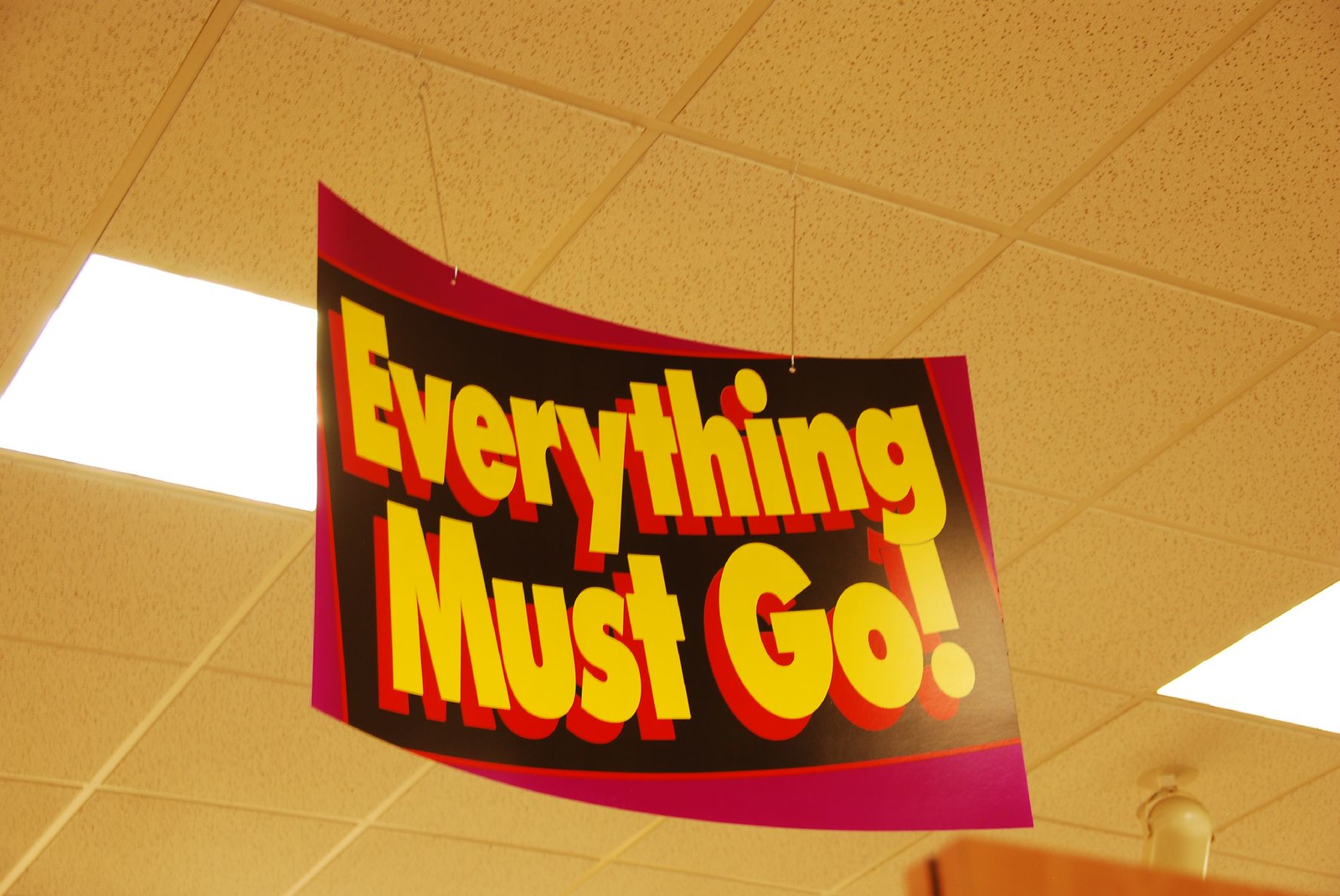This close-up photograph captures the interior of a retail store, focusing primarily on the ceiling elements. The ceiling is composed of white tiles, with fluorescent lighting casting a slightly yellow hue across the scene. Prominently featured in the image is a rectangular sign hanging from the ceiling, brightly colored in yellow, red, and hints of purple. The bold yellow font on the sign declares, "Everything Must Go!" in an urgent tone, emphasizing a clearance or sale event.